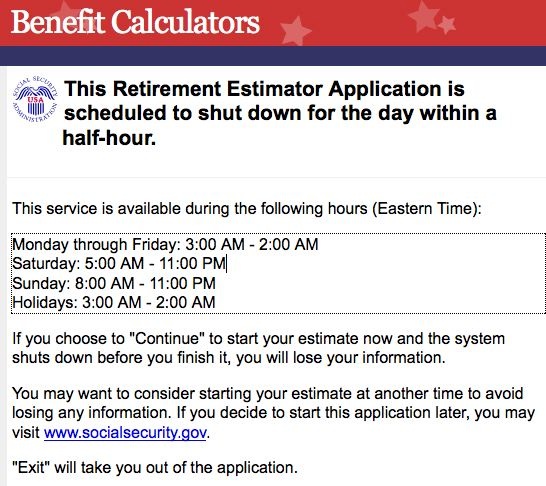The image is a screenshot of a webpage, likely viewed on a laptop, desktop, smartphone, or tablet. The webpage features a distinct red bezel at the top, with the text "Benefit Calculators" prominently displayed in bold white letters. Faded stars subtly embellish the background, adding a patriotic touch. Below this, a blue band spans the width of the screen. 

Dominating this section is a blue American Eagle emblem, complete with a shield that bears the "USA" inscription in red letters, adding to the patriotic theme. Beneath the eagle, various blue bands are displayed. 

The main body of the message is in bold black text, informing users that "This retirement estimator application is scheduled to shut down for the day within a half hour." Following this, in somewhat smaller bold text, the operational hours are listed: 

- Monday through Friday: 3 AM to 2 AM (Eastern Time)
- Saturday: 5 AM to 10 PM
- Sunday: 8 AM to 11 PM
- Holidays: 3 AM to 2 PM

There is a small space followed by a warning stating, "If you choose to 'continue' to start your estimate now, and the system shuts down before you finish it, you will lose your information." Another space follows which advises, "You may want to consider starting your estimate at another time to avoid losing any information. If you decide to start this application later, you may visit" with the hyperlink, "www.socialsecurity.gov", provided for easy access. Finally, a prompt to "exit" the application is included, indicating it will take the user out of the current estimator tool.